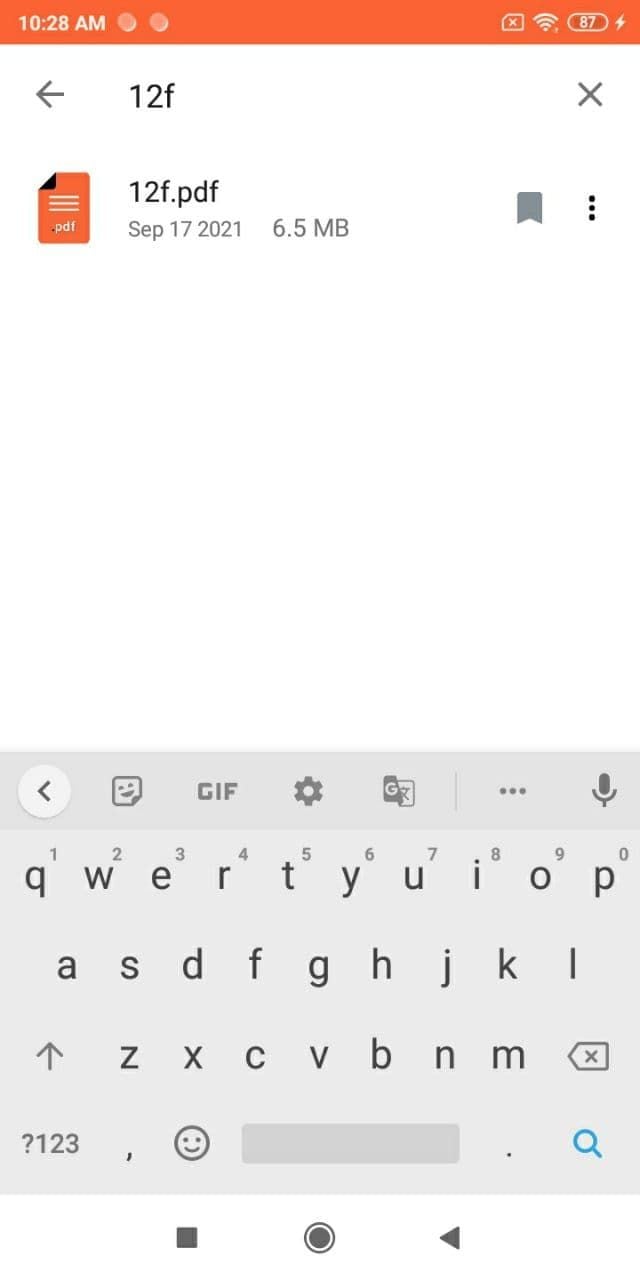A detailed screenshot from a smartphone showcases various interface elements and features:

At the very top of the screen, the time is displayed as "10:28" in white, followed by two dots on the right side. Moving to the far right, the battery life is indicated as "87%", and it is currently charging, as evidenced by the lightning bolt symbol. The entire taskbar at the top is highlighted in orange.

Beneath the taskbar, on the far left, there is a left arrow icon. Adjacent to this arrow, the text "12F" is displayed. On the far right of this section, there is an "X" icon, presumably for closing or exiting the view.

Below this top navigation area, there is a PDF file titled "12F," which was created on September 17, 2021, and has a file size of 6.5 megabytes. An option to bookmark this file is available, but it is currently not activated, indicated by a grayed-out bookmark icon. To the right of the bookmark icon, three vertical dots are stacked, suggesting additional options or settings.

Between the PDF description and the back button, there is a large, blank space. Below this space is a gray keyboard interface. This keyboard includes an option to hide it by clicking the left arrow at the top row. To the right of this arrow is an emoji button. Continuing to the right, there is a button for GIFs, which allows users to browse and select various animated images or videos, ranging from humorous to serious content.

Additional buttons on the keyboard include a settings button, a voice-to-text option, and the standard layout of letters. At the bottom of the keyboard, users can switch between numbers, symbols, traditional emojis, and a search function.

Overall, the screenshot captures a comprehensive view of the smartphone's user interface, highlighting various navigation and functional elements.